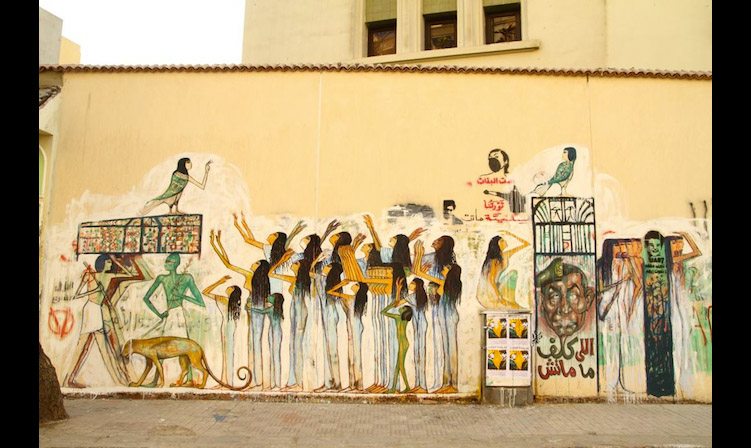The photograph captures a vibrant and detailed mural painted on an outdoor wall. The mural, set against a cream-colored backdrop, features numerous elements that draw from ancient Egyptian iconography as well as modern graffiti art. 

Starting from the left, there is an Egyptian man walking from left to right, followed by a leopard and another Egyptian man painted in blue. Above these figures, there's a depiction that may represent a casket or a cabinet. Atop this object sits a mythical creature, likely an Egyptian deity, portrayed as a half-bird, half-human figure, adorned in shades of black, green, and cream.

On the ground beneath this scene, a group of eight to ten women dressed in whitish-blue gowns stand raising their arms towards the bird-person deity, seemingly in an act of worship. To the right of these women, a seated woman is depicted with her leg up and her hand resting on her head, adding to the narrative dynamic of the mural.

Further right, modern graffiti art intersects with the ancient motifs. There's a detailed graffiti portrait of a man's face with expressions suggesting he is wearing a black face covering. Above this, another bird-person figure is seen, adding consistency to the thematic elements of the mural. Adjacent to this portrayal is a graffiti-style depiction of a green and black zombie-like figure, linking the contemporary vibe with the historical artwork.

The scene is brightly lit, with the clear daylight enhancing the vivid colors which range from greens, blues, browns, and beiges to blacks and reds. Visible in the top left corner is a bright sky, contrasting with a tall, beige building in the background. The bottom portion of the image shows a clean sidewalk, indicating that the mural is located in an outdoor urban environment. The overall clarity and lighting give the photograph a crisp, clear appearance, highlighting the detailed and eclectic mix of historical and modern artistic styles.